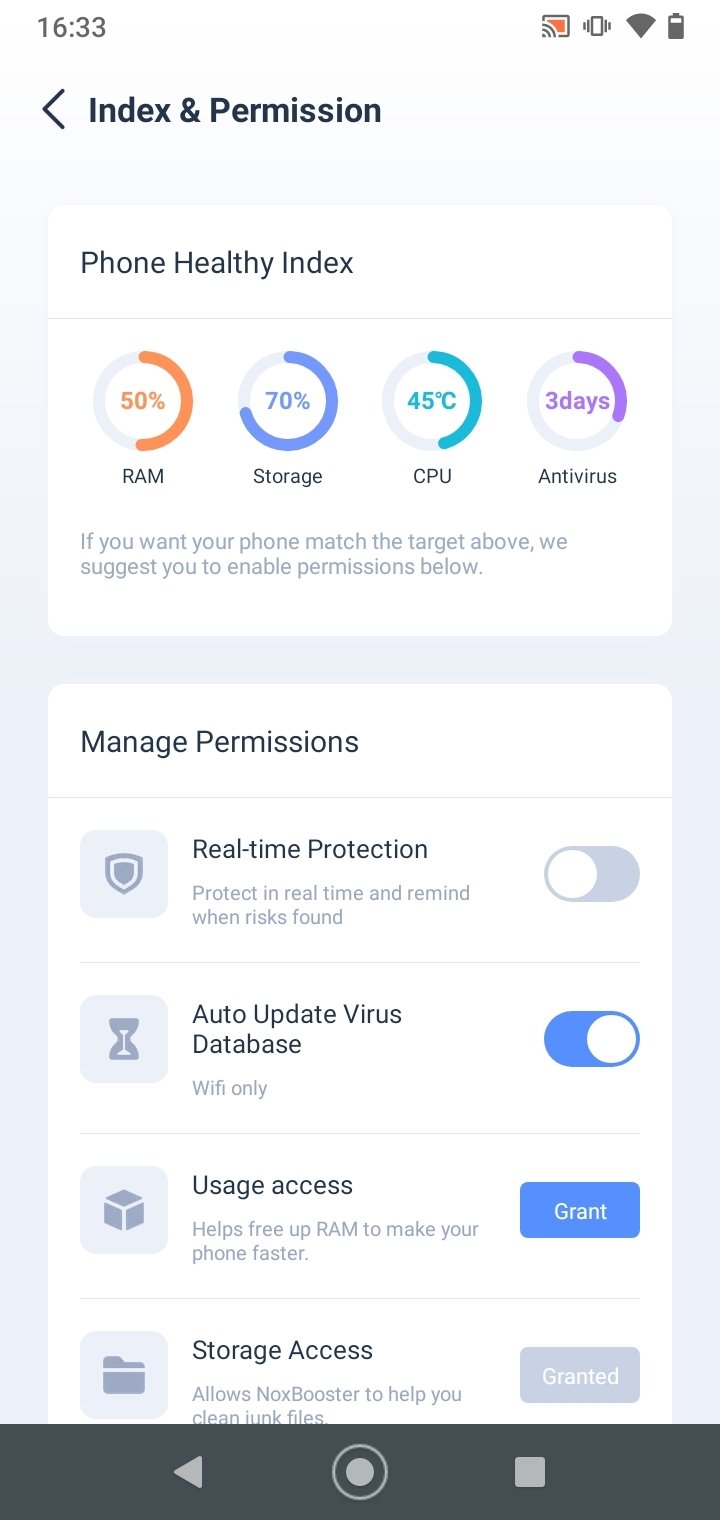This image is a screenshot from a mobile phone, capturing the top portion of a webpage. The screenshot includes the standard phone interface elements, such as the time displayed as 16:33, indicators for WiFi strength, and battery percentage. 

Beneath these status indicators, the webpage title "Index and Permission" is prominently displayed in large black text with a left-pointing arrow next to it. The page presents a "Phone Health Index" section, which visually depicts various performance metrics: RAM usage at 50% indicated in orange, storage at 70% shown in blue, CPU temperature at 45°C marked in blue, and antivirus status labeled "Three days" in purple.

Below these metrics is a recommendation text suggesting users enable permissions to match the targeted performance above. There's a "Manage Permissions" section listing four categories: "Real-Time Protection," "Auto-Update Virus Database," "Usage Access," and "Storage Access," each accompanied by representative icons—a shield, a clock, a 3D box, and a folder, respectively.

The current status of these permissions is also displayed: "Auto-Update Virus Database" is enabled, "Real-Time Protection" is disabled, "Usage Access" has a blue activation button to the right, and the "Granted" button for "Storage Access" appears blurred out.

At the bottom of the screenshot, the phone's navigation buttons are visible: the back button shaped like a triangle, the home button as a circle, and the recent apps button represented by a square.